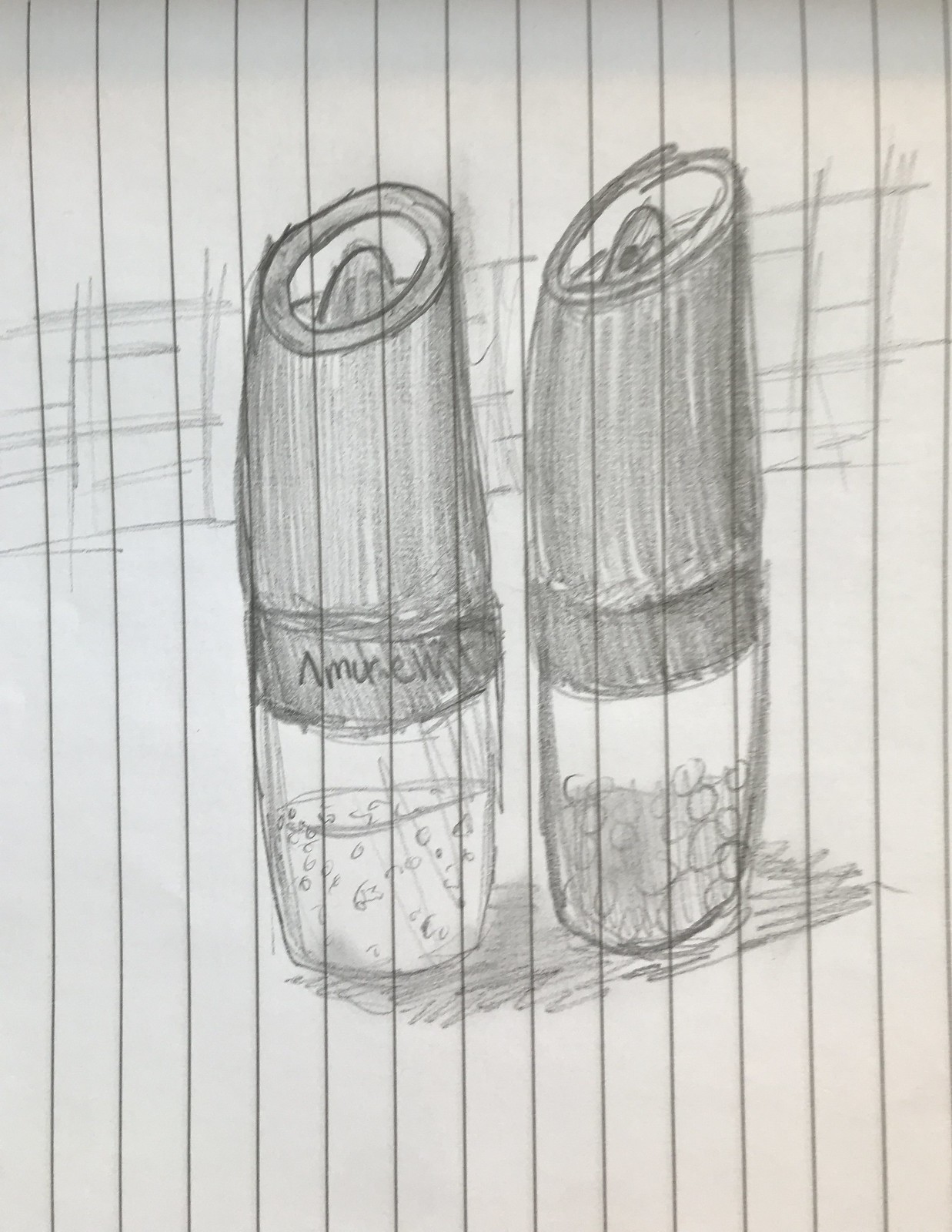A detailed pencil drawing on vertically lined notebook paper showcases two spice bottles with prominent grinders on their tops. The bottle on the left, identified as a salt shaker, contains small clear crystals, while the bottle on the right, a pepper shaker, is filled with larger black circles representing peppercorns. Both bottles feature intricate cross-hatching near their tops, darkening these areas. There's some indistinguishable text on the salt shaker, possibly reading "ammo" or "amaranth." The sketch includes scribbles suggesting shadows beneath the bottles and subtle background cross-hatching implying a wall, although no actual surface is drawn. The entire image is rendered in shades of white and gray.